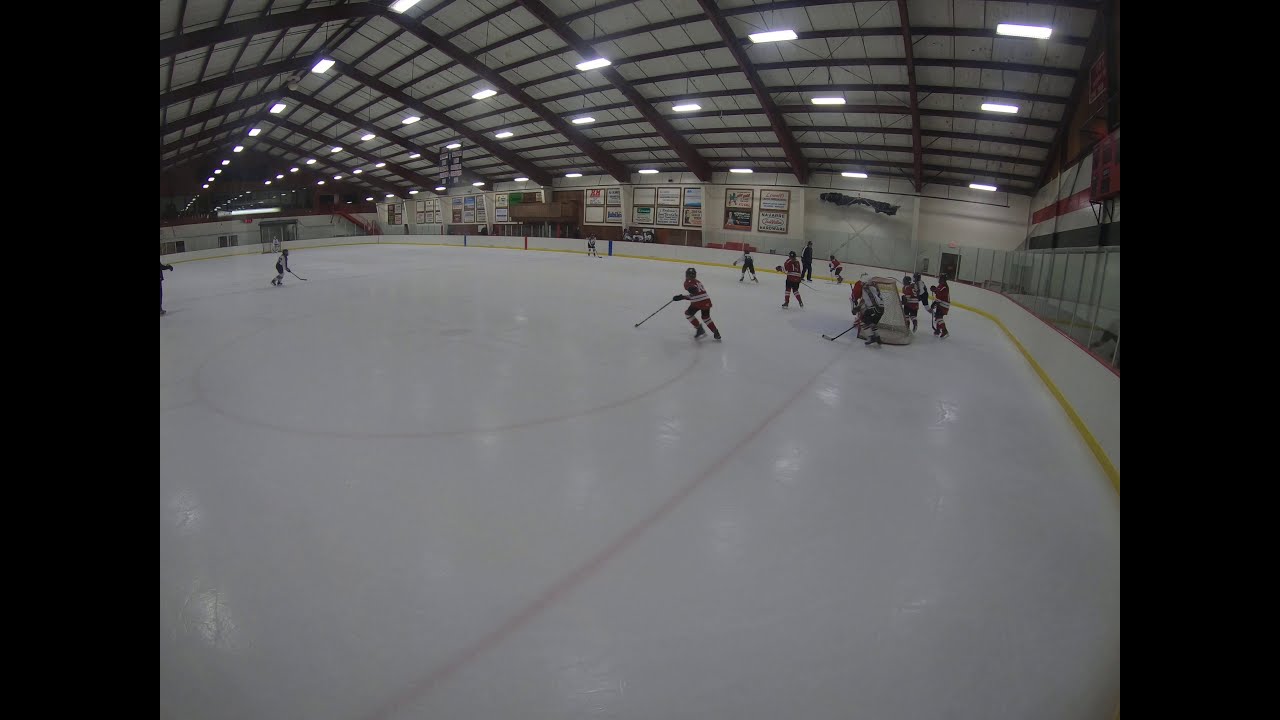The image captures a dynamic scene inside a large indoor hockey rink and auditorium. The arena features a grid-patterned ceiling with dark brown support beams and white metallic panels, from which rows of glowing fluorescent lights hang, illuminating the space below. The walls are white with a gray bottom trim, adorned with an array of banners, flags, and possibly awards or championship posters, adding a sense of history and accomplishment to the venue.

On the pristine white ice rink, two teams are engaged in a lively hockey game. One team sports red and black uniforms, while their opponents are dressed in white and black. Multiple referees in traditional black and white attire skate around, overseeing the match, with a goalie visible far in the distance guarding the net. The rink's perimeter is defined by a solid yellow line, enhancing visibility.

Additionally, black rectangles frame the image from the left and right, contributing to the photo's structured composition. Despite the bustling activity, the environment appears more recreational than professional, as indicated by the absence of spectator stands or bleachers. An exit sign, red-railed steps, and doors are also visible, indicating the points of egress in the facility.